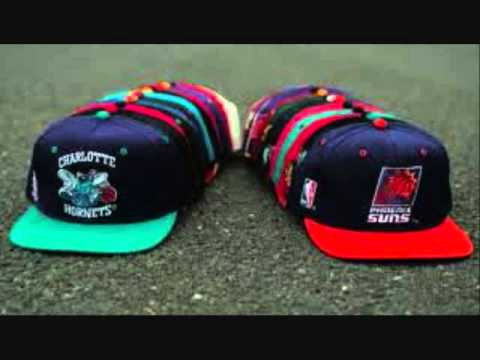The image showcases two rows of baseball caps meticulously lined up on a grayish, asphalt-like surface, possibly a display or a store setting. Each row features a series of caps stacked together, extending back at least eight to ten deep. The caps are all of the same style, featuring a variety of colors, but prominently displaying team logos.

On the left row, the foremost cap is primarily blue with a teal brim and bears the inscription "Charlotte Hornets" along with the team's logo on the front. This cap has a distinct dot at the top and ventilation holes strategically placed—two in the front and two on the sides. The caps behind it reveal a spectrum of colors including black, red, light blue, purple, and beige.

To the right, the leading cap is dark blue with a bright red brim, marked with the Phoenix Suns’ name and a red graphic within a square. Additionally, this cap features the NBA emblem on its left side. As the caps recede into the background, they slightly converge, touching each other in the distance but spaced apart at the front.

The image is framed with a thick border at both the top and bottom, highlighting the depth and colorful variety of the baseball caps arranged in neat rows.